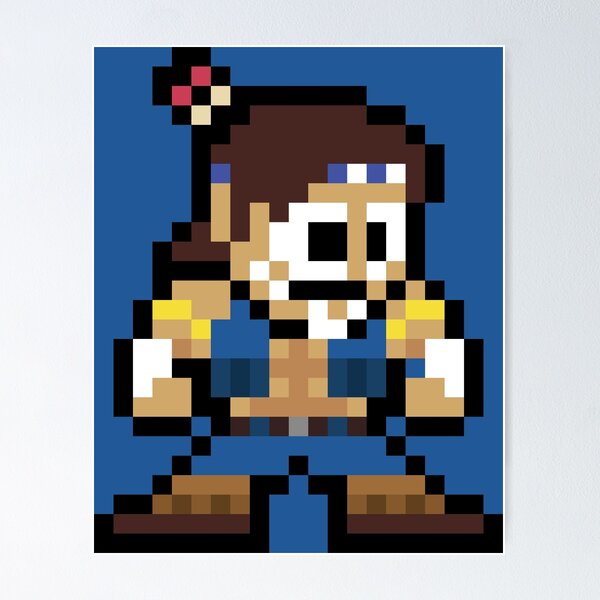The image features an 8-bit pixelated character reminiscent of a Mega Man-style graphic set against a blue background. The figure is composed of distinctly blocky squares, each color taking up a pixel in typical 8-bit fashion. The character's attire suggests a Native American theme, with a blue and white headband and what appears to be a red feather protruding from his brown hair. He sports a blue vest left unbuttoned, exposing his bare chest, and blue pants or perhaps shorts, complemented by brown shoes. His facial features include black, wide eyes, and potential facial hair, though the pixelation makes it difficult to discern finer details. The character's arms show small white patches near the wrists and a gold line near the shoulders, adding to the intricate detailing despite the up-close and highly pixelated nature of the graphic.